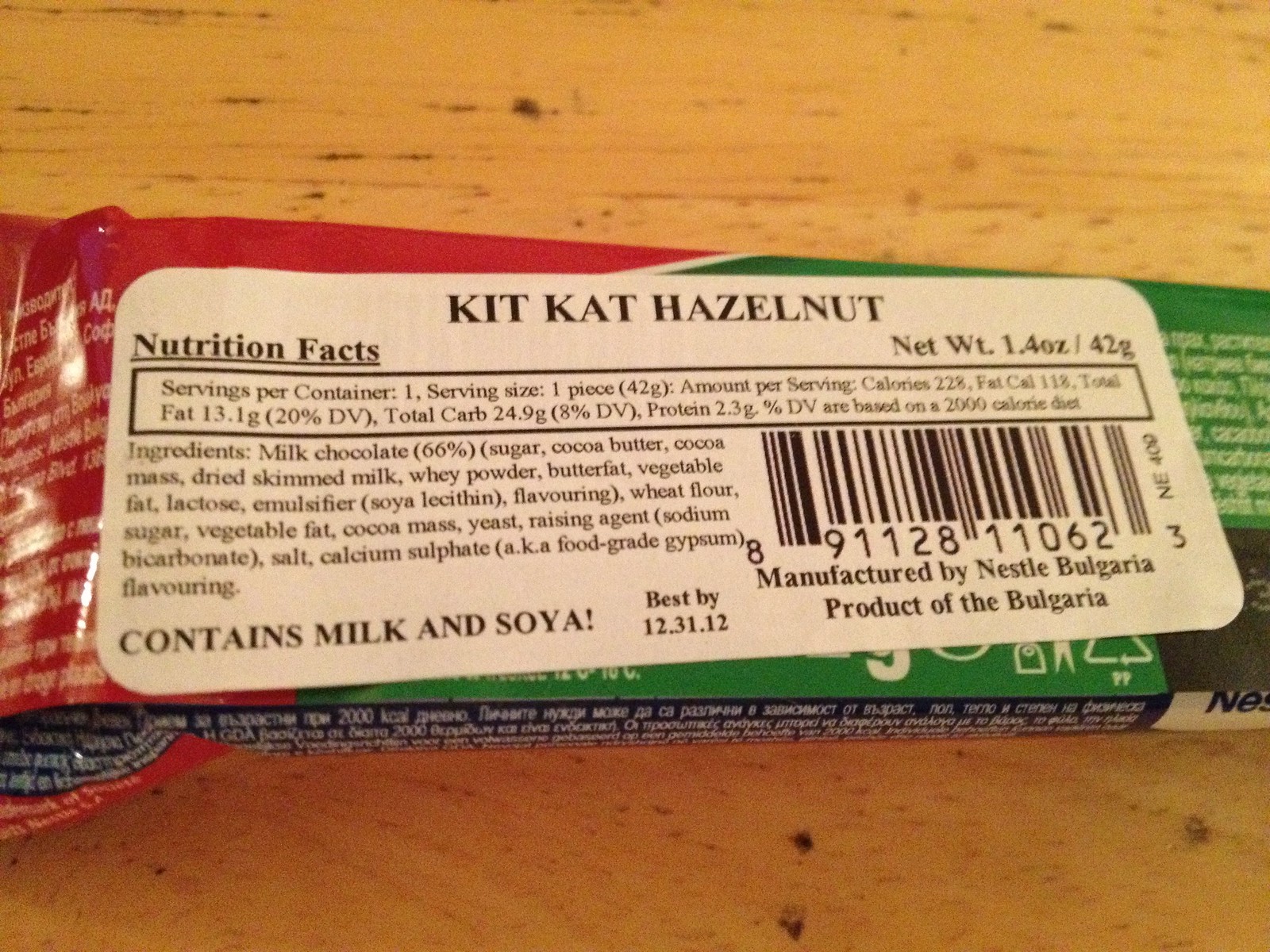The image depicts the nutrition facts on the back of a packaged bar, which is lying on a medium-toned wooden surface, showcasing the intricate brown details in the grain. The bar is wrapped in a plastic packaging with a distinct color scheme: predominantly red on the left side and green on the right side. A bluish strip runs along one edge of the packaging. The product is identified as being manufactured by Nestle, as indicated at the bottom of the packaging. The white label in the center is rectangular with rounded edges. At the top of this label, in black text, it reads "KitKat Hazelnut." The nutrition facts state that one serving provides 228 calories, and the net weight is 1.4 ounces (42 grams). Additionally, the label notes that the bar contains milk and soy and is a product of Bulgaria, manufactured by Nestle Bulgaria. The ingredients listed include milk chocolate, wheat flour, sugar, vegetable fat, among others.